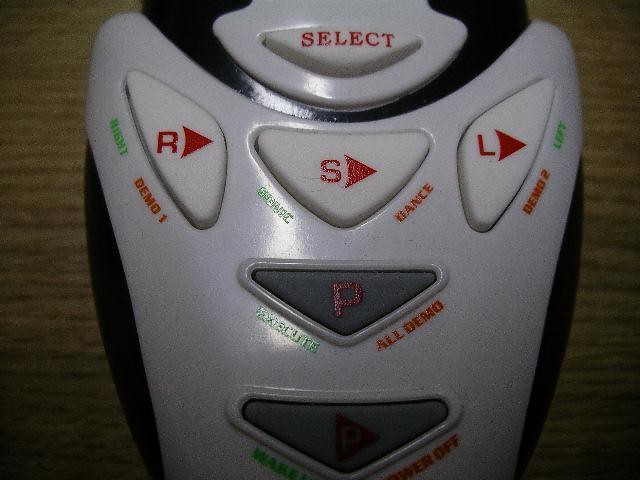This color photograph captures a remote control predominantly featuring a white center with black edges. The topmost part of the remote showcases a triangular button labeled "Select" in red letters. Below this, a row of three white triangular buttons is arranged horizontally. The left button displays a red “L” with a right-facing triangle and is labeled "Demo 2" and "Left" in red text. The middle button bears a red "S" inside a right-facing triangle and is labeled "Dance" in red text, with some green text that's not clearly visible. The right button has a red "R" with a right-facing triangle, and it is marked "Right" in green and "Demo 1" in red text. 

Below this central row, there are two black triangular buttons. The top black button is marked with a red "P" and is labeled "All Demo" in red text, and the bottom black button contains a white "P" inside a red triangle facing downward, accompanied by the words "Demo Off." The remote is placed on a wooden surface, providing contrast to its detailed and colorful design.